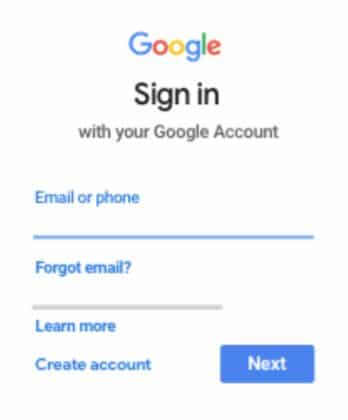The image depicts a login page for Google. Located at the top center, the iconic Google logo is displayed, featuring a capital "G" in blue, a lowercase "o" in red, a second lowercase "o" in yellow, a lowercase "g" in blue, a lowercase "l" in green, and a lowercase "e" in red. Below the logo, the phrase "Sign in" is prominently shown in large black letters, followed by the tagline "with your Google Account" in smaller gray text, with both "Google" and "Account" capitalized.

To the left, in a small Arial-like font, the instructions "Email or phone" are written in blue. Below this is an editable text field, outlined in light blue to indicate that it is currently selected. Further down, the link "Forgot email?" is displayed in blue, providing an option for users who need help retrieving their account information. Another gray, non-editable text field follows, suggesting its temporary disabled status.

Beneath this, the text "Learn more" appears in blue, indicating a clickable link for additional information. The phrase "Create account" is also presented in blue and is clickable.

To the right side of the image, there is a clickable rectangular button with rounded edges, containing the word "Next" in bold white text. The overall image quality is fuzzy, particularly affecting the smaller text above the editable fields and the "Next" button, giving the impression of a low-resolution screenshot.